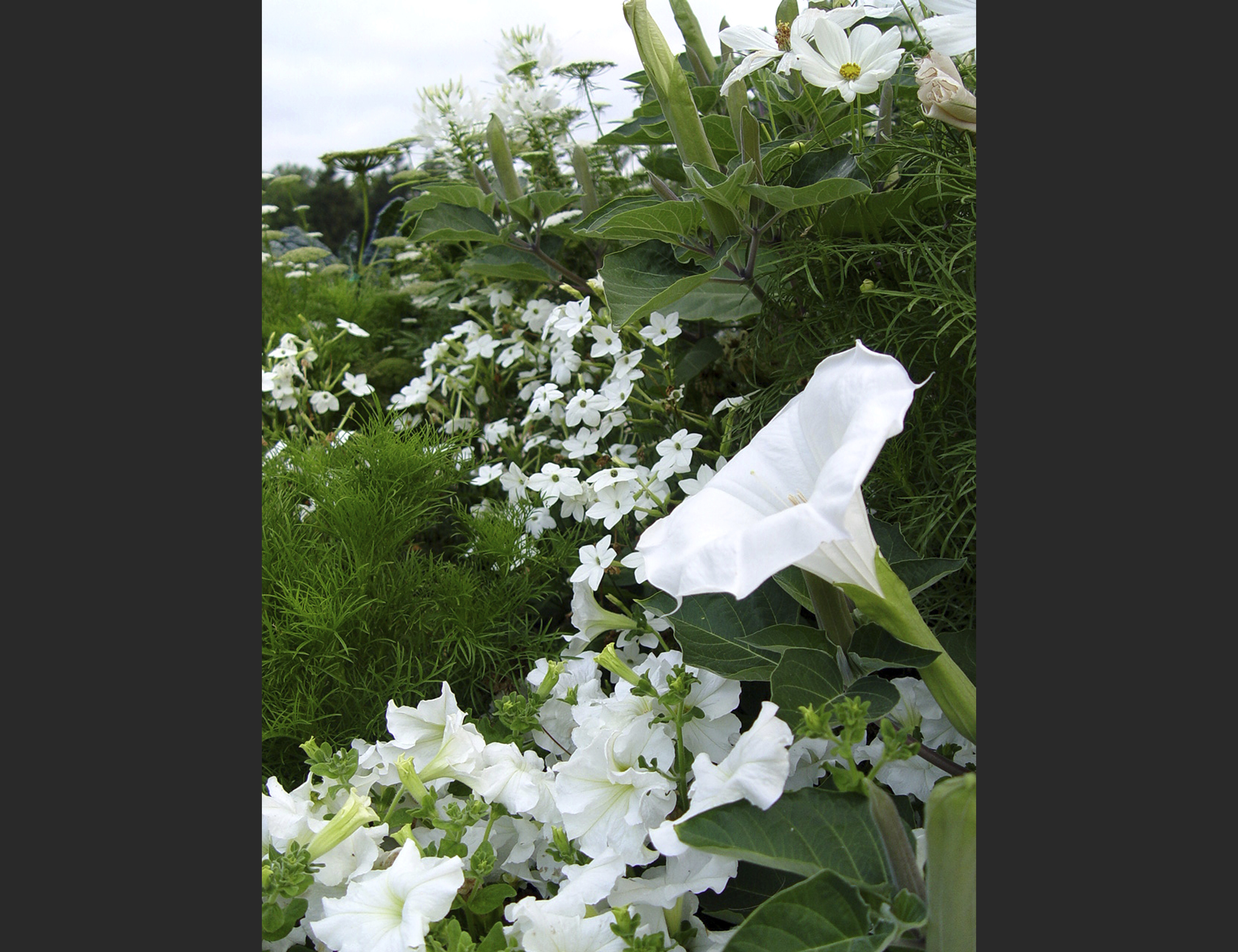This close-up, vertically cropped photograph immerses you in a snippet of nature teeming with lush greenery and various white flowers. Dominating the foreground on the right is a prominent, bell-shaped white lily, exuding elegance. Surrounding the lily are multiple types of white flowers, including open and closed white daisies positioned in the corners of the image. These blooms are interspersed among a dense array of green plants and foliage, extending upwards and filling the scene with vibrant life. In the background, a cloudy, light-gray sky hints at an overcast day, adding contrast to the vivid whites and greens. The photo’s sides are marked by dark gray borders, emphasizing its cropped and slightly dark, bluish tone. The combination of flowers, greenery, and the faintly visible sky creates a dynamic, natural composition.